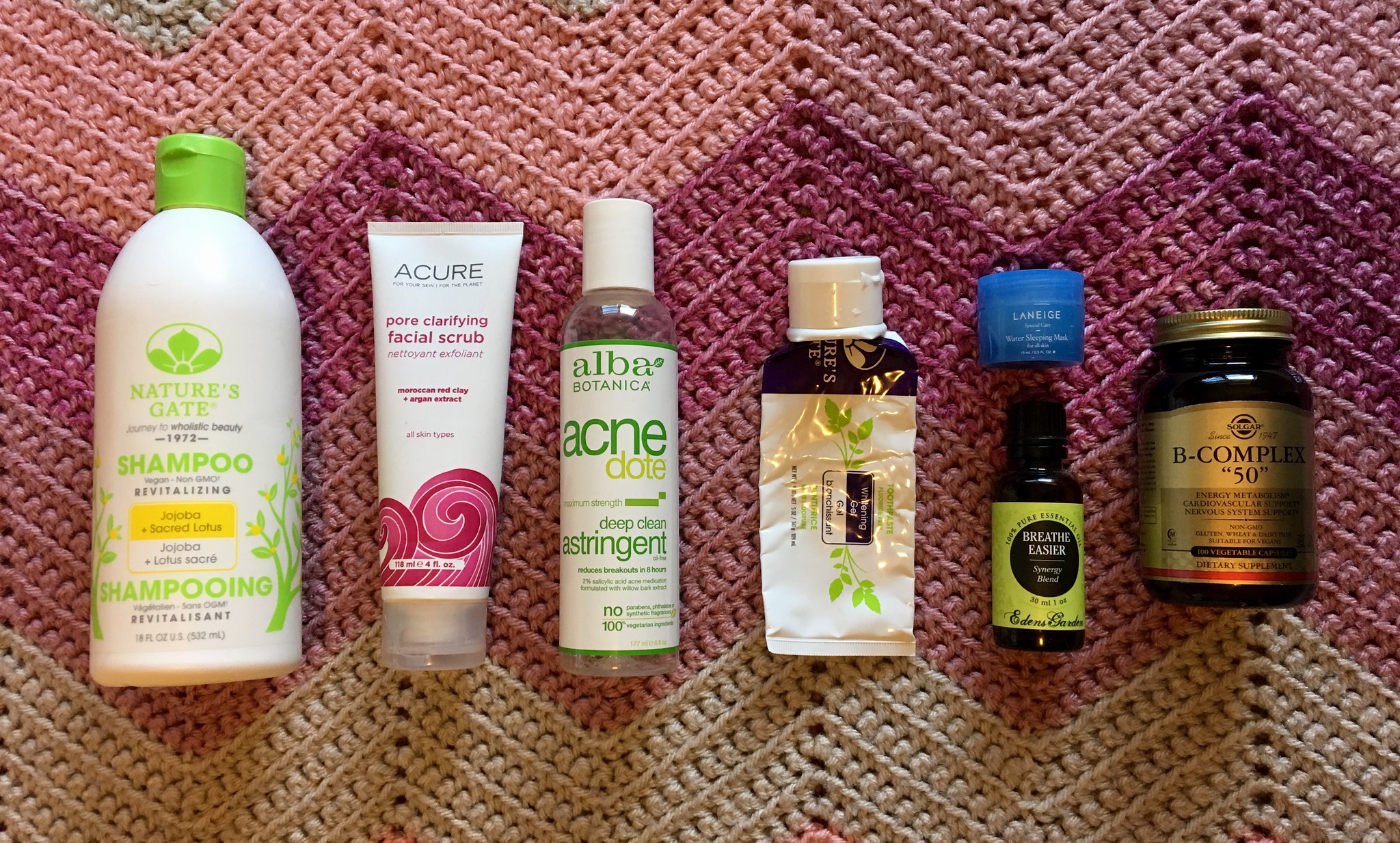The color photograph captures a collection of beauty products and supplements meticulously arranged on a crocheted blanket. The close-up display showcases a section of the blanket adorned with a zigzag pattern in shades of pink, lavender, purple, another pink hue, and white, creating an ombré effect. The image is presented in landscape orientation, allowing for a detailed view of the products.

From left to right, seven distinct items are visible:

1. **Nature's Gate Shampoo**: A white plastic bottle with a green cap. The bottle features integrated graphics in green, yellow, and black font.
   
2. **Acure Clarifying Facial Scrub**: A white squeeze tube adorned with pink and red swirls at the base, complemented by a translucent screw-on cap.
   
3. **Alba Botanica Acnedote Deep Clean Astringent**: A clear bottle with a white screw-on cap and a labeled design primarily in white and green with some yellow lettering.
   
4. **Unidentified Product**: An almost empty, squished foil tube with a white flip-cap. The tube is decorated with green lettering and leaves.
   
5. **Breath Eraser**: A tiny medicine bottle, possibly containing peppermint drops or tincture, though the exact contents remain unclear.
   
6. **Lancôme Jar**: A small blue screw-top jar, likely containing a skincare product, though the label is difficult to read.
   
7. **B Complex 50 Supplement**: A jar with a brass or gold-colored screw-top lid, indicating a vitamin supplement.

The arrangement on the crocheted blanket with its vibrant and soothing pattern juxtaposes the practical, everyday nature of the beauty and wellness products, creating an aesthetically pleasing composition.